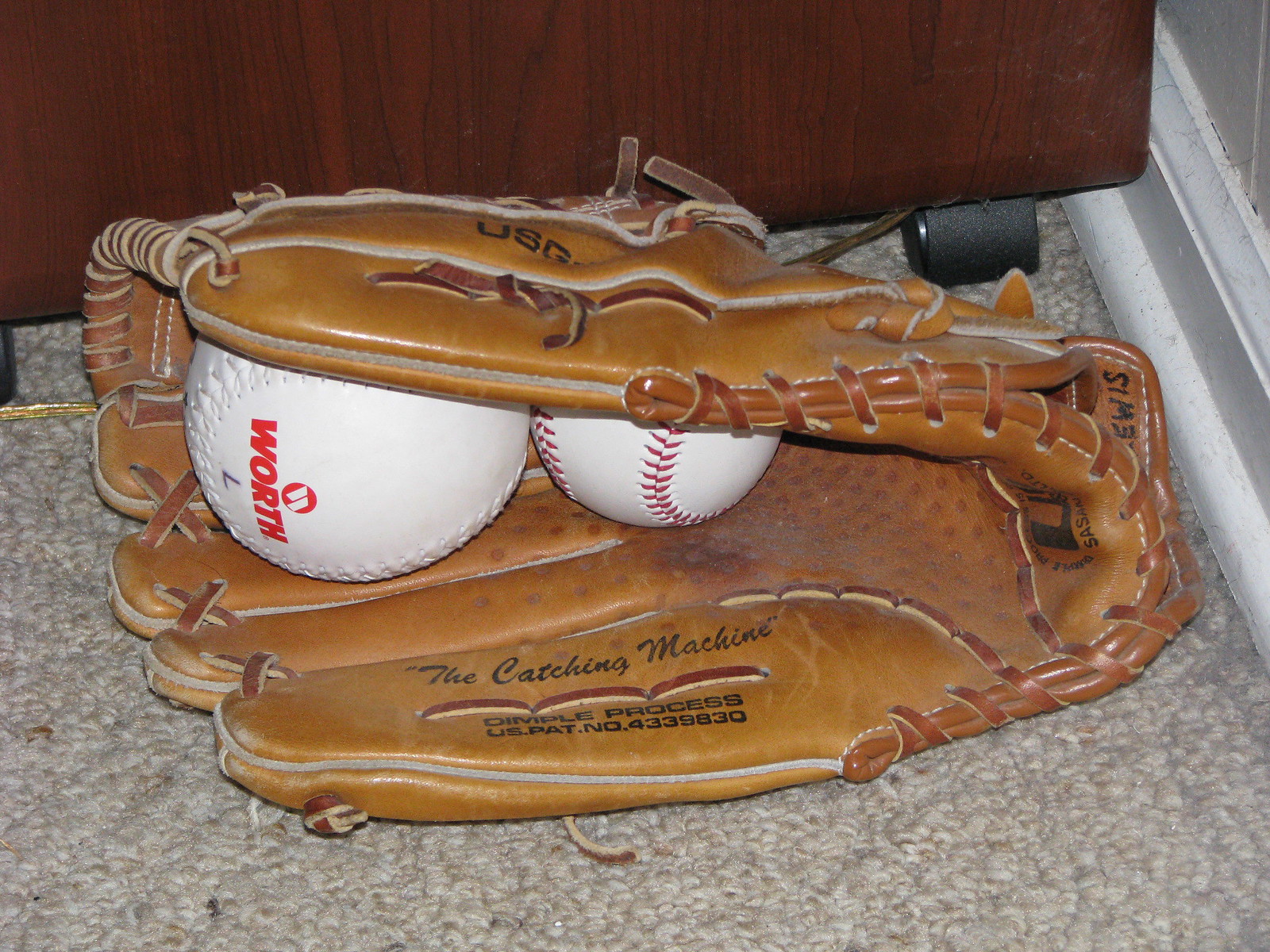This photograph captures an overhead view of a classic brown baseball mitt, lying on a gray textured carpeted floor. The mitt, featuring darker brown stitching, showcases a broken-in, well-loved appearance. It holds two balls: a larger white softball with the brand name "Worth" in red, and a standard white baseball with red stitches. Within the mitt, the text "The Catching Machine" is visible, along with a patent number, and the top displays the initials "USG." Additionally, the glove bears a handwritten marker inscription "ICEWIS," likely part of someone's name. The scene includes a brown wooden cabinet on black caster wheels, situated against a wall adorned with a somewhat dirty white baseboard trim, adding context to the room's setting.